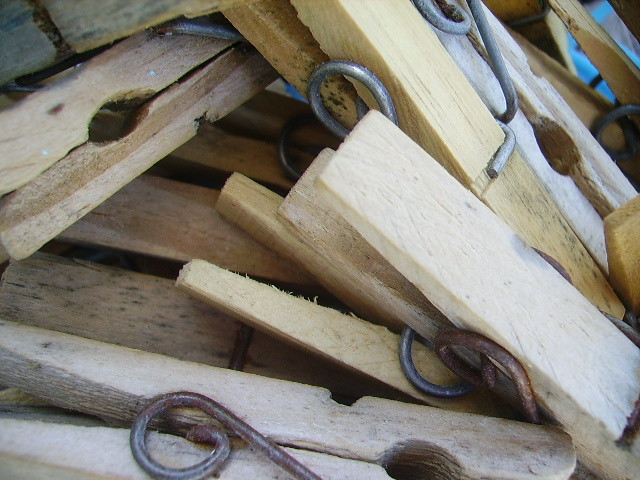The image depicts a collection of wooden clothespins piled together, primarily light to medium brown in color. Each clothespin features a metal spring coil, some of which show slight rust. The texture and appearance of the wood vary, with some pieces displaying split edges and knot holes. Amongst the clothespins, there appear to be metal objects with curled ends, akin to hangers. The scene is likely captured during daylight. Additionally, there are three blue objects scattered in the upper part of the image, the exact nature of which is unclear. Overall, the photograph captures the rustic, slightly worn nature of the wooden clothespins and their metallic components, all gathered closely in one area.